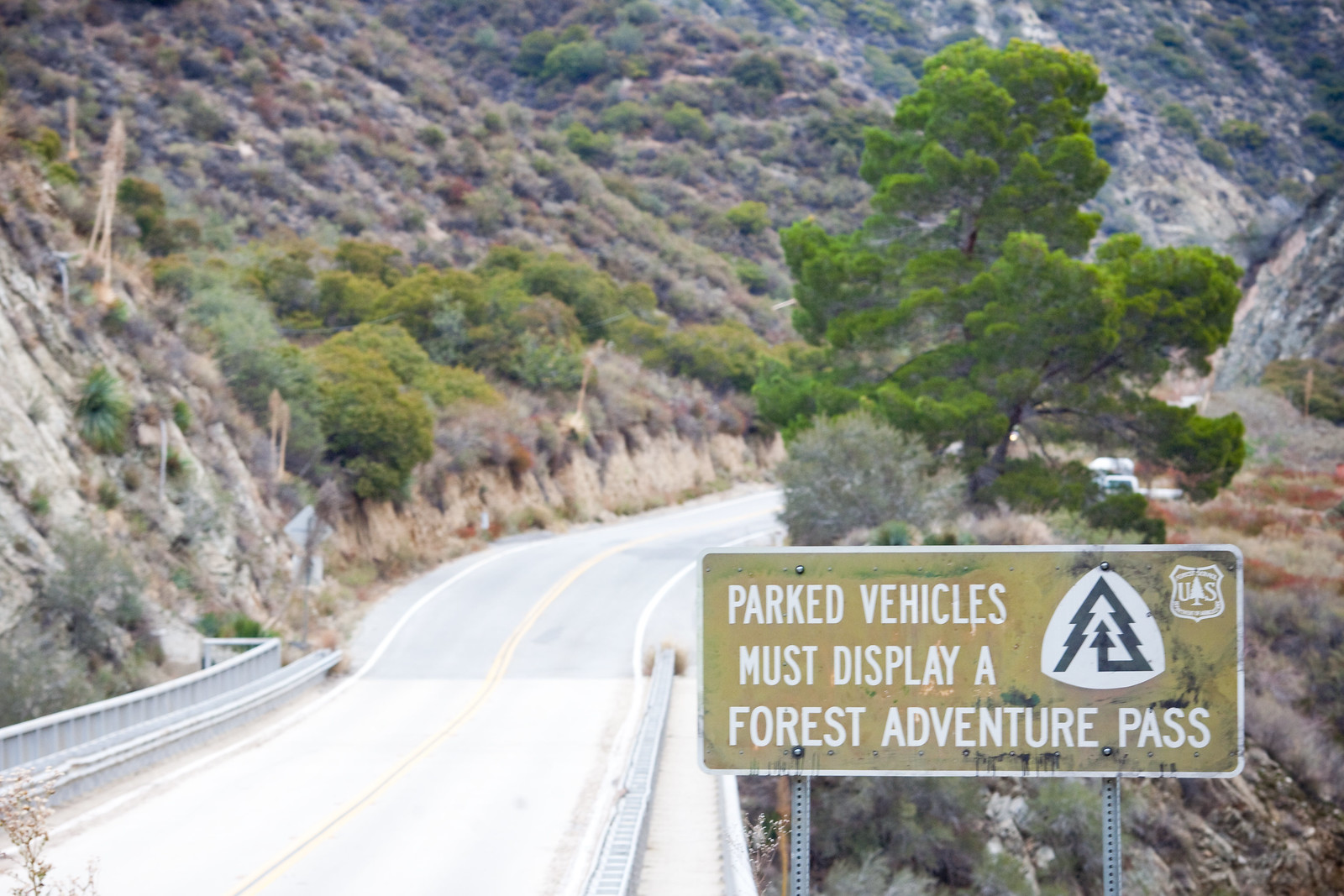This photograph, seemingly an older and slightly grainy daytime image, captures a two-lane road cutting through a steep canyon with rocky cliffs and sparse vegetation. As the road enters a grey steel bridge, marked by light grey paving and guardrails, its coloration darkens, aligning with a double solid yellow line down the center and single white lines marking the edges. On the right-hand side of the road, beneath a prominent green pine tree, several cars are parked. The setting is dry and rocky with dead plants scattered around. A brown rectangular sign with white text, positioned on metal posts in the lower right-hand corner, reads "Parked Vehicles Must Display Forest Adventure Pass," with a white shield above displaying a tree logo in black and a triangular badge inscribed "U.S. Forestry." The left side of the image is characterized by a steep hillside covered with trees, bushes, and hedges, contrasting the barren, dry hills on the right.